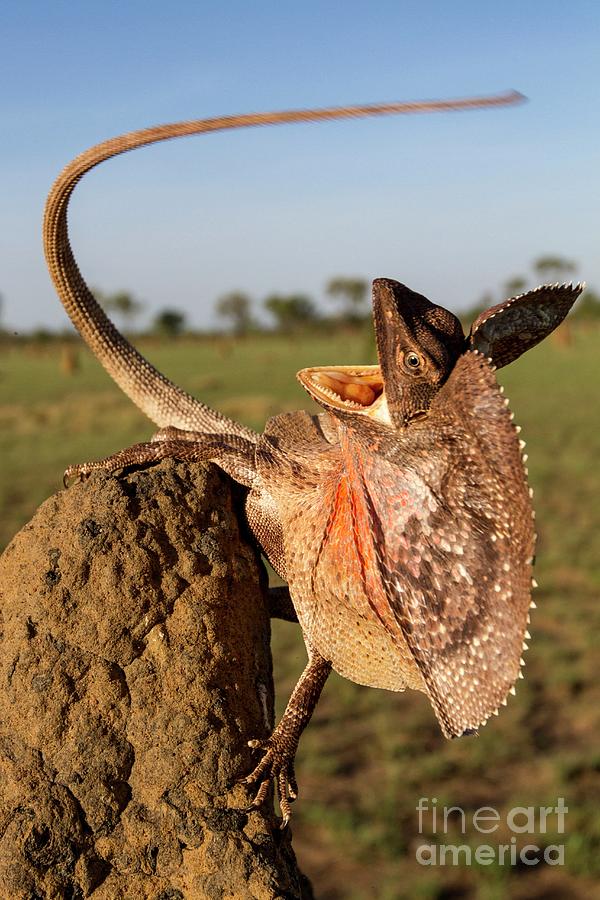The photograph captures an intense moment of a frilled-necked lizard perched atop a vertically narrow, jagged rock structure, its mouth wide open in an aggressive stance, possibly mid-roar or hunting. The lizard, primarily brown with pale white spots, an orangish underbelly, and a reddish-orange interior of its mouth, has a long, thin tail that curves dynamically behind it, partially out of focus, indicating swift movement. This fine-scaled lizard appears to have a frilled neck tinged with yellow, tan, and hints of pink or orange. Its small, beady eyes add to its fierce demeanor, while spikes running down its back enhance its reptilian appearance. The photograph is set outdoors on a sunny day under a gradient sky that transitions from a darker blue at the top to a lighter gray-blue near the horizon, which is lined with trees and a patch of green, somewhat brown-tinged grass. The brand name “Fine Art America” is subtly positioned in the bottom right corner, with 'Art' and 'America' bolded. The background is artistically blurred, drawing the viewer's focus to the dramatic and detailed presentation of the lizard.